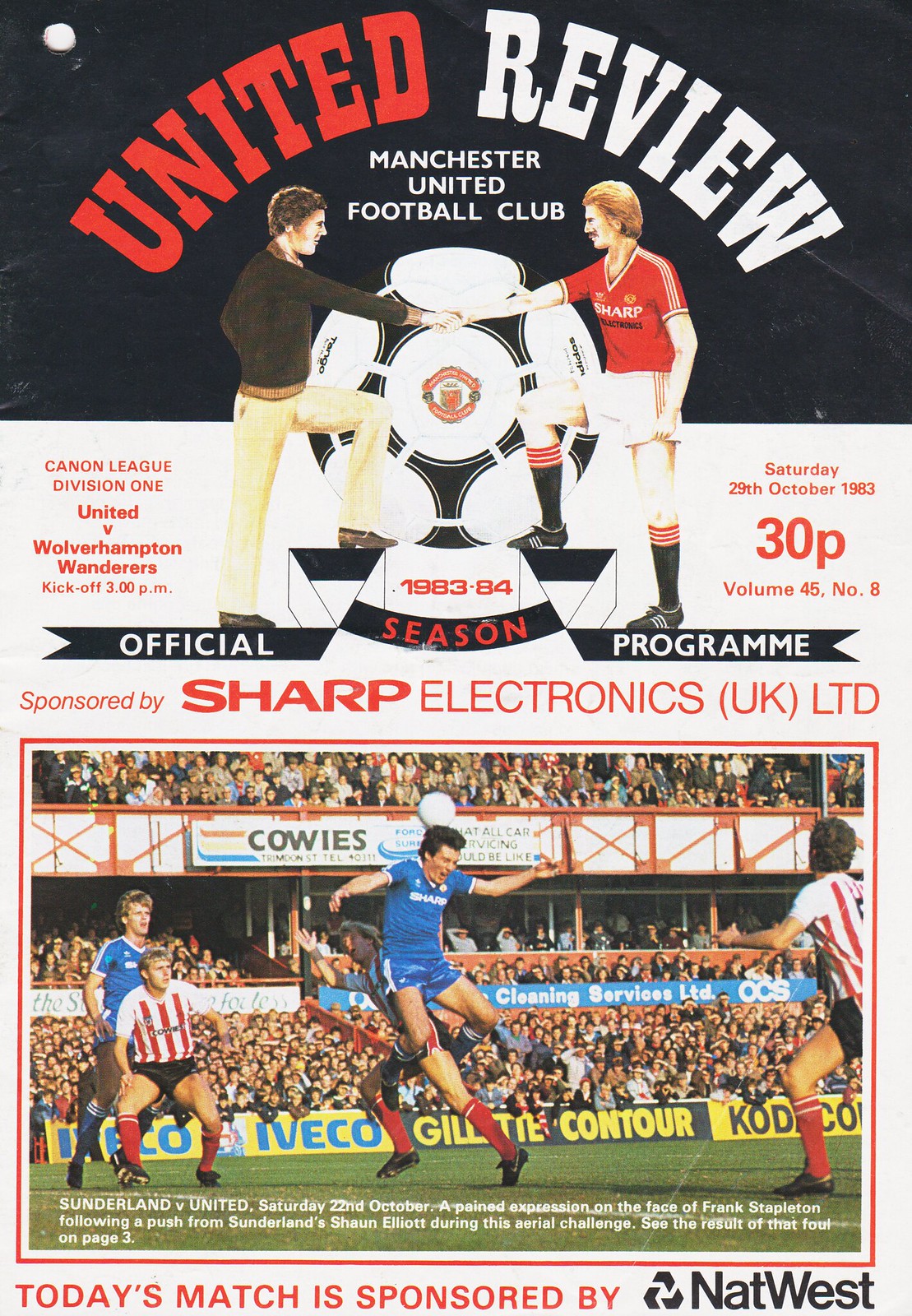The image showcases an official program from the Manchester United Football Club for the 1983-84 season. At the top, on a black background, the title "UNITED" is emblazoned in red, followed by "REVIEW" in white. Directly underneath, in white lettering, it states "Manchester United Football Club." Below this heading, there is a drawing depicting two soccer players shaking hands in front of a soccer ball. The player on the left sports khaki pants and a black sweater, while the player on the right is dressed in a red and white soccer uniform with black shoes.

Further down, the program indicates the years "1983-84" and labels itself as the "OFFICIAL PROGRAM." Just below this, in red lettering, it proclaims, "SPONSORED BY SHARP ELECTRONICS, UNITED KINGDOM LIMITED." 

The bottom half features a vivid color photograph capturing a real-life soccer match, with players donning either blue or red and white uniforms. Beneath this action shot, additional white text narrates a particular moment: "Sunderland v. United, Saturday, 22nd, October. A pained expression on the face of Frank Stapleton following a push from Sunderland's Sean Elliott during an aerial challenge. See the results of that foul on page three." At the very bottom, it notes, "TODAY'S MATCH IS SPONSORED BY NAT WEST."